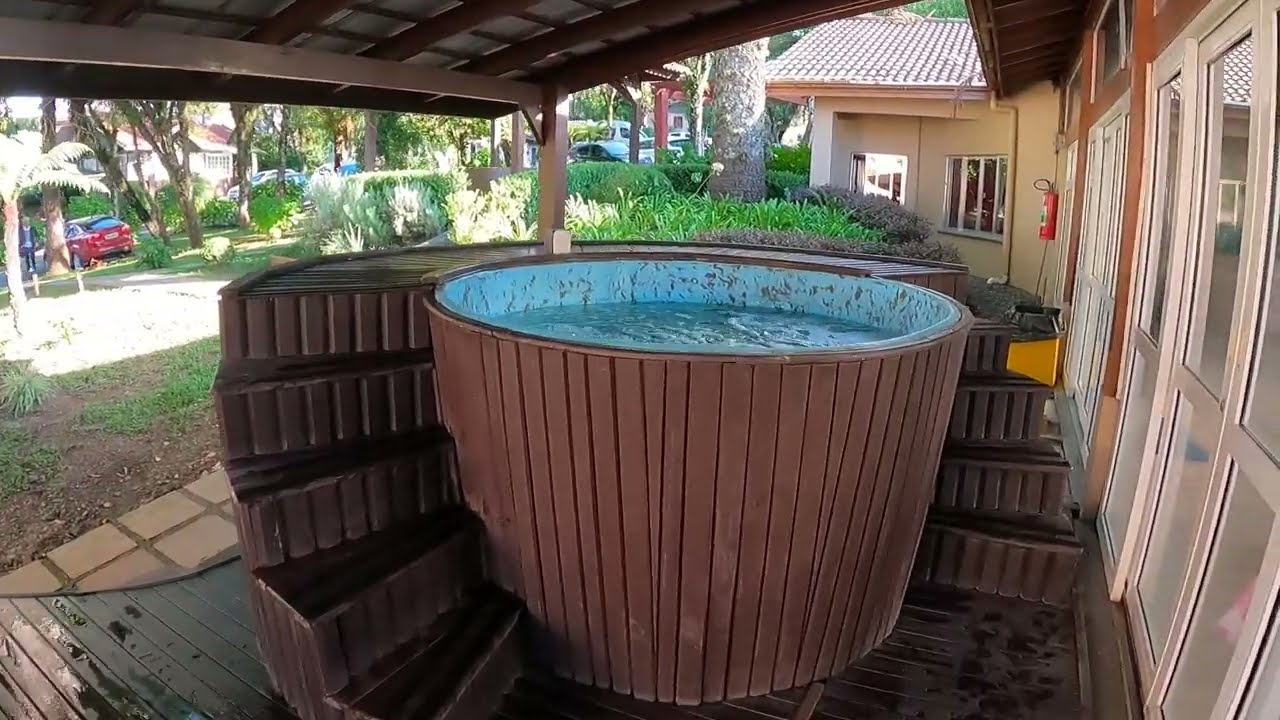The image captures a detailed outdoor scene centered around a circular, wood-paneled hot tub situated in what appears to be a retreat or resort-like area. The hot tub features vertical brown wooden slats and is filled with light blue water. Surrounding the hot tub are brown wooden steps leading up to a platform designed for easy access. The setting is under a veranda, supported by silver metal beams and brown wooden support structures, with a brown decking floor.

Adjacent to the hot tub is a light brown building with numerous silver and glass doors and windows framed in white. This building may be a part of a larger resort complex, implied by the presence of palm trees and lush greenery in the background, along with multiple parked vehicles, including a prominently visible small red sedan and other cars. The area feels like an inviting retreat with its distinct design elements, such as a stone path transitioning into a grass yard on the left and a red fire extinguisher mounted on the building wall. Additionally, the ground surrounding the hot tub area is shiny, suggesting it has been recently wet, likely due to the presence of bathers.